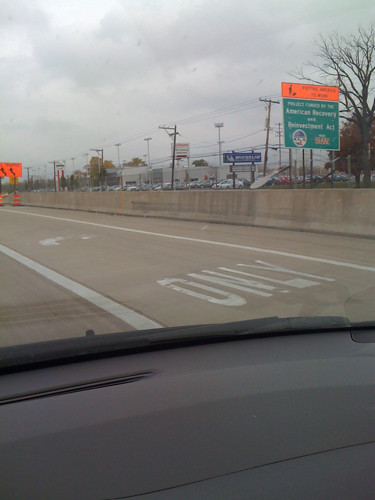The image depicts a view from the driver's side of a vehicle's dashboard. The scene outside appears to be taken on an overcast day, characterized by the presence of numerous gray clouds. A set of electrical lines can be seen traversing the sky. There's a prominent, green, boxy directional sign mounted on poles, topped by a smaller red sign providing additional information. Indications of the fall season are evident as one of the visible trees is devoid of leaves. A concrete guardrail lines the side of the road, extending into the distance until it meets another sign. This secondary sign seems to indicate a change in road direction, suggesting a slight veer to the side.